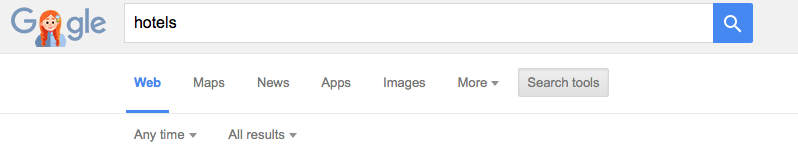This is the home page of a website featuring a minimalist and clean design. The top inch of the page is light gray, creating a subtle header area, while the rest of the background is predominantly white.

In the top left corner, the website features a distinctive logo: a cartoon girl resembling the Wendy's character, with long orange braids draped over her shoulders. She has a small flower on the right side of her head, matching orange eyebrows, large brown eyes, and expressive black pupils. She wears a shirt with a dark blue left side and a light blue right side to complete her look.

To the right of the logo is the website's name displayed in bold, lowercase letters, starting with a 'g' followed by 'l' and 'e'. Adjacent to this is a prominent search bar that extends to within an inch of the right margin. Inside the search bar, the term "hotels" is pre-typed in black lettering. At the far right end of the search bar, there's a blue square containing a white magnifying glass icon, signifying the search function.

Below the search bar, aligned under the word "hotels," is a navigation menu with options starting with "web" in blue, underlined, then followed by options: "maps," "news," "apps," "images," and "more" in black, with "more" featuring a drop-down tab. To the right of these options, there's a gray tab labeled "search tools" in black lettering.

Directly beneath this menu, a thin gray line spans the width of the page, providing visual separation. Under the "web" option in the navigation menu, two additional options are displayed in black: "anytime" with a drop-down tab, and "all results" with a drop-down tab. The remainder of the page is mostly empty white space, occupying approximately two-thirds of the image's height, contributing to a clean and uncluttered aesthetic.